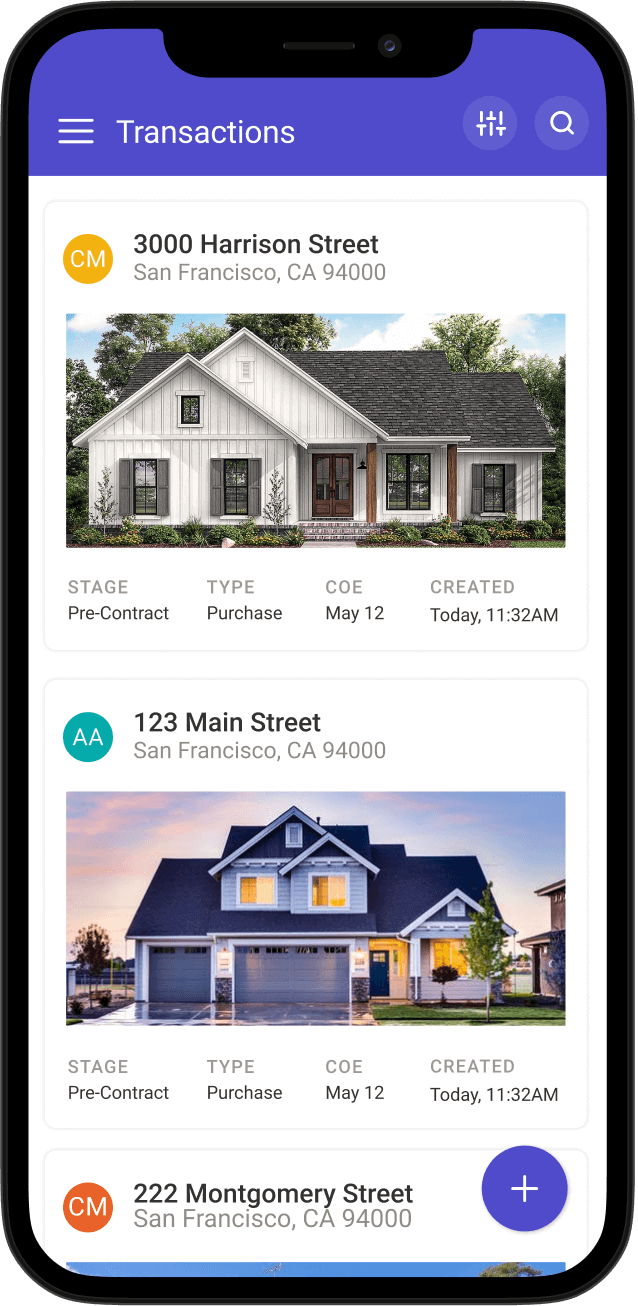A detailed screenshot of a smartphone display, primarily focusing on a housing website. The image showcases the following elements:

The smartphone has a black, rectangular frame with rounded corners. At the top, there's a small, curved black area housing a front camera lens on the right side. Below this, the screen background is a gradient shade of purple.

### Top Navigation Bar:
- **Left Side:** Three horizontal lines, commonly known as the hamburger menu icon, in white.
- **Middle:** The word "Transactions" in white, with a capitalized 'T'.
- **Right Side:** Two circles with a slightly lighter purple shade. The right circle features a white outline of a magnifying glass, while the left circle has an icon resembling a vertical 'I', an upside-down 'T', and a lowercase 't'.

### Main Section:
A white background serves as the primary area, presenting a list of properties for sale, each including detailed address information and corresponding images.

1. **First Property:**
   - **Address:** 3000 Harrison Street, San Francisco, CA 94000
   - **Icon:** A yellow circle with 'CM' in white lettering.
   - **Image:** A single-level ranch house with a shingle gray roof, trees, and shrubs in the background. Blue sky with white clouds are visible. Features include two front windows, a peak roof window, a brown double front door, and several additional windows.
   - **Details:**
     - **Stage:** STAGE (in gray)
     - **Status:** PRE-CONTRACT (black, capital P and C)
     - **Type:** TYPE (gray) - PURCHASE (capital P)
     - **COE:** COE (gray) - MAY 12
     - **Created:** CREATED (gray) – Today at 11:32 AM

2. **Second Property:**
   - **Address:** 123 Main Street, San Francisco, CA 94000
   - **Icon:** A green circle with 'AA' in white lettering.
   - **Image:** A two-level or possibly single-level house with a gray roof. Features include a three-car garage with a large door and a smaller door, windows indicating possible upstairs bedrooms, shiny driveway suggesting recent rain, and landscaped grass with a small tree. Another house is partially visible on the right side. The sky is light blue with pink clouds, hinting at early morning or afternoon.
   - **Details:**
     - **Stage:** STAGE (gray)
     - **Status:** PRE-CONTRACT (black), capital P and C with a dash in between.
     - **Type:** PURCHASE (capital P)
     - **COE:** MAY 12
     - **Created:** Today at 11:32 AM

3. **Third Property:**
   - **Address:** 222 Montgomery Street, San Francisco, CA 94000
   - **Icon:** An orange circle with 'CM' in white lettering.
   - **Additional Element:** To the right, a purple circle with a white plus sign.
   - **Image:** Only the top of another image is visible, showing a blue sky and a small tree in the right upper corner.

Overall, the screenshot provides a cohesive look at listings and relevant details such as address, status, and time of creation.